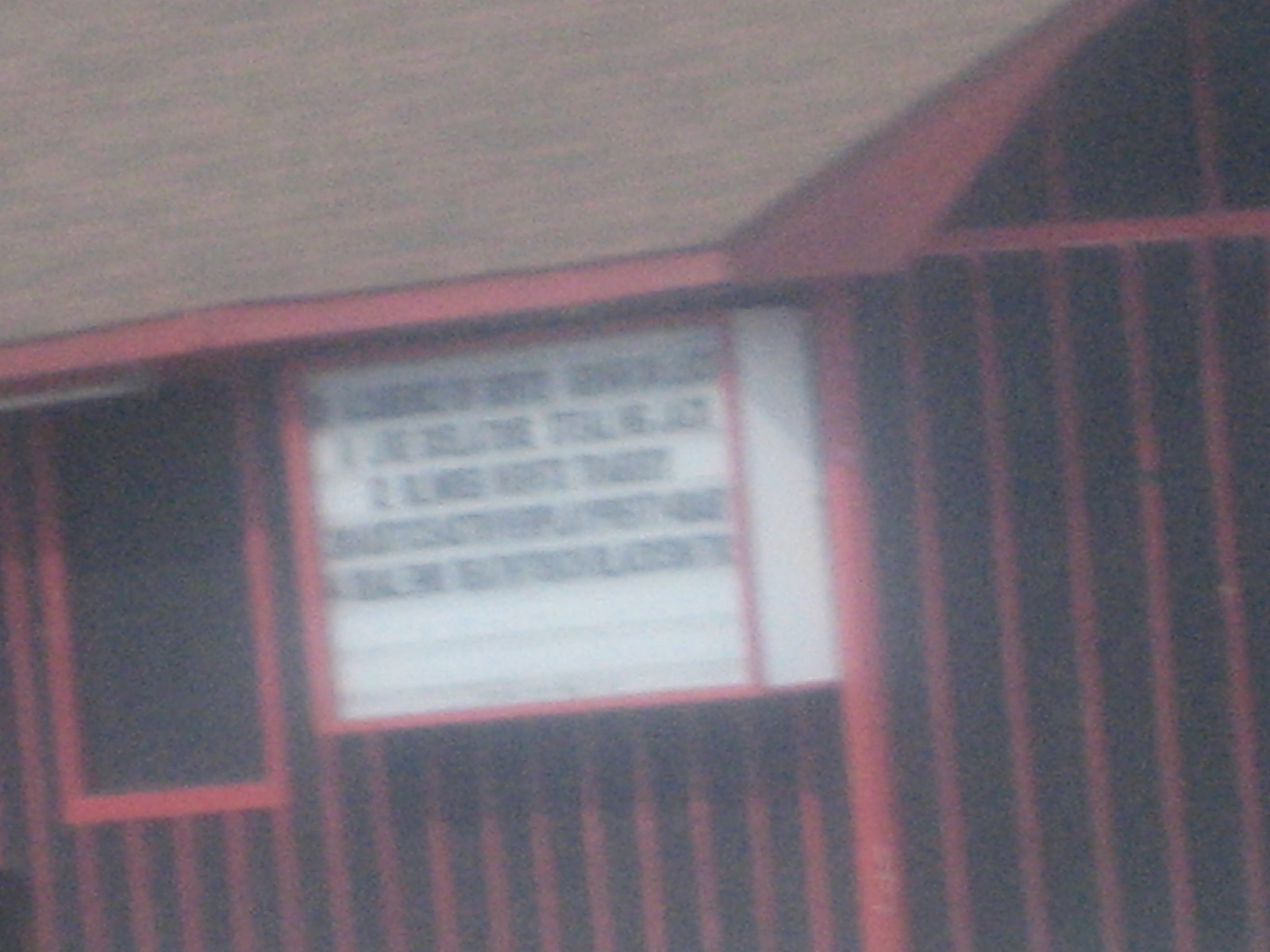This photograph captures an enigmatic exterior of a building, which might be a restaurant or a church. The structure is painted black with distinct red stripes, and features a red brick roof that slopes upward to an unseen peak. A prominent white marquee billboard adorns the building, though its text is largely unreadable due to the image’s graininess and artifacts. What is legible includes black lettering listing various items or events, with identifiable entries like "1" and "2," where the second entry appears to mention "Ladies Night" and a fragment that resembles "Therapy." The overall blurriness makes it challenging to discern the building's exact purpose or the details on the billboard.